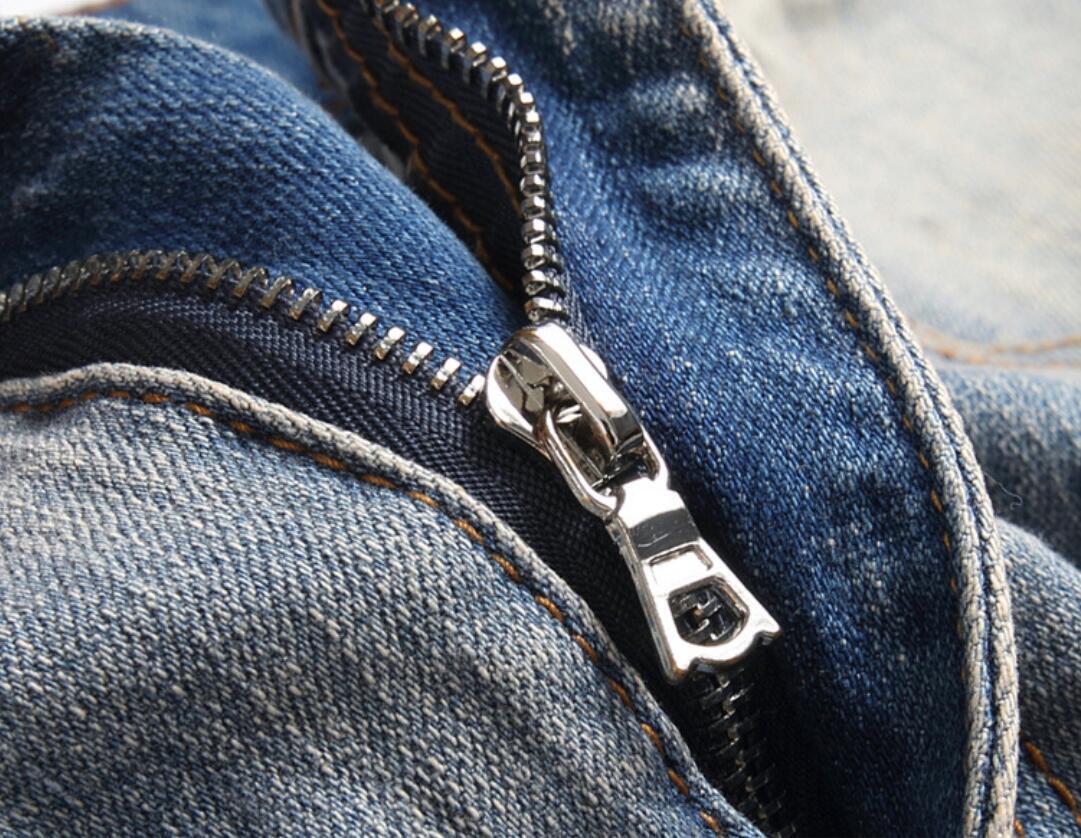This is a highly detailed close-up photograph of a partially unzipped metal zipper on a pair of denim jeans. The silver, high-quality zipper is prominently featured at the center of the image, with its shiny teeth clearly visible. The zipper is positioned about halfway down. Surrounding the zipper, the denim fabric is a mid-blue shade, exhibiting signs of wear, with lighter, more faded patches revealing some white threads. A flap of the jeans, pushed aside to the right, exposes a less worn, darker navy blue interior. The brown seams in the denim, sewn with brown cotton thread, are visible and appear to be of high construction quality. In the background, the upper right corner contains a small area of cream color, while the rest of the image is dominated by the various hues and textures of the denim material.